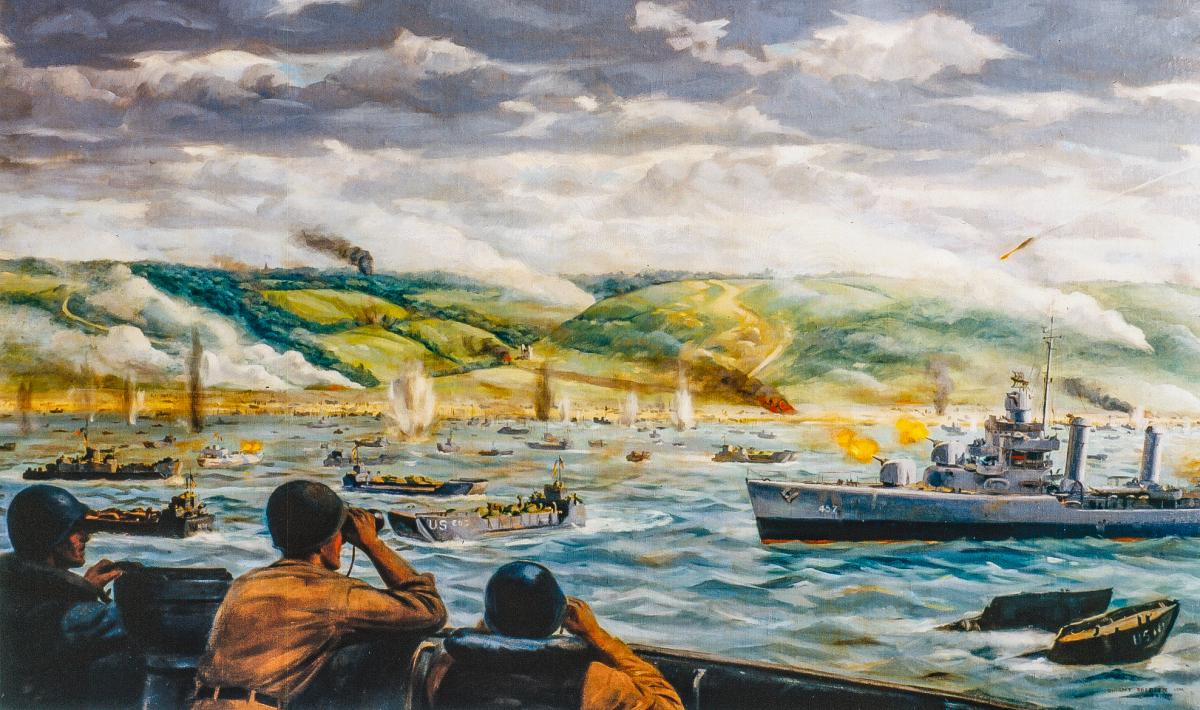This painting vividly portrays a dramatic naval battle scene. At the heart of the tumultuous ocean filled with choppy waves, a fleet of warships, including an imposing aircraft carrier and several naval vessels, engage in fierce combat. The atmosphere is chaotic, with guns blazing from the aircraft carrier and frequent explosions erupting both in the water and on a nearby hillside, sending plumes of smoke into the air. In the foreground, a boat carrying three soldiers, fully outfitted in combat gear and helmets, cuts through the waves as the men peer through their binoculars, assessing the battlefield. The overcast sky adds a somber tone to the intense and gripping scene.